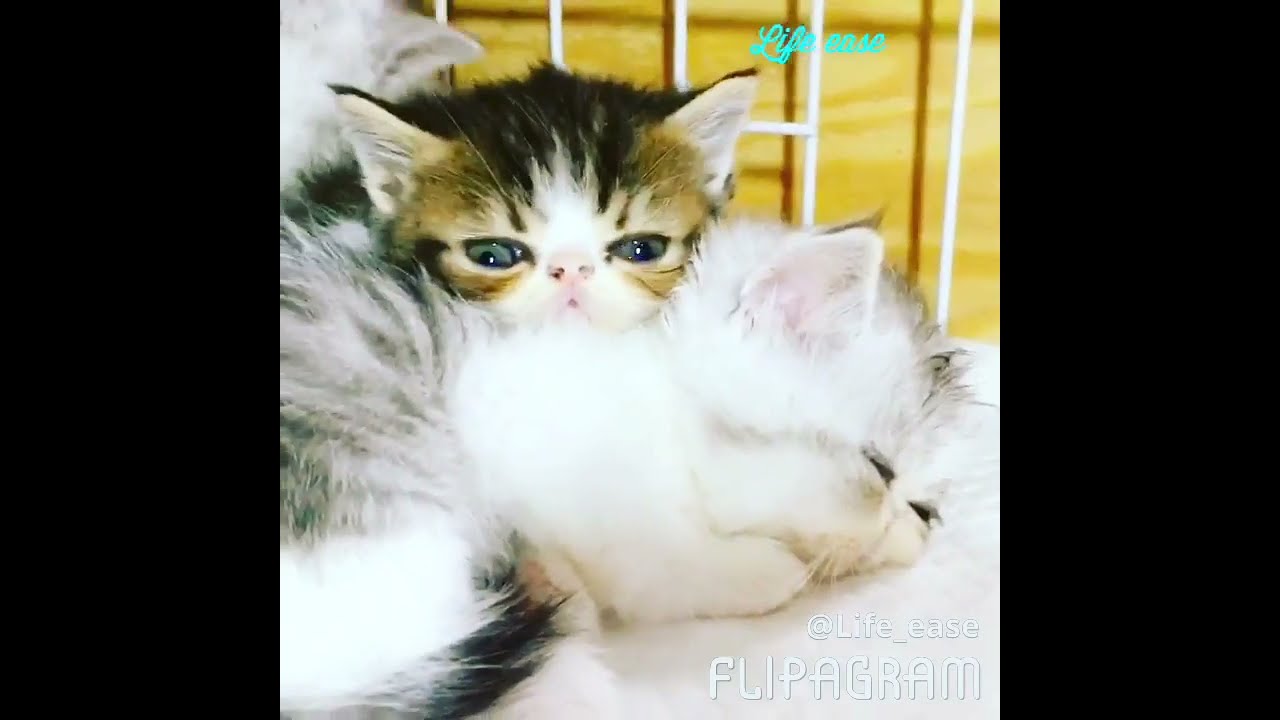This photograph captures an indoor scene featuring two adorable kittens in close contact. One kitten with predominantly dark brown and black fur, accentuated by beige hues and an adorable pink nose, is resting atop another kitten. The kitten underneath, who is primarily white with subtle gray streaks and touches of brown and black, appears to be half-asleep with his eyes partially closed. Both kittens exhibit a sense of calm while lying on a soft, white fabric surface. In the background, there is a metallic white fence with a yellow wall behind it. The image bears the watermark "@life_is_flipagram" in the bottom right corner, and the word "Life" is written in small blue cursive letters in the top right corner. Adding to the charm, part of a third kitten's head, which appears to be white and gray, is visible in the upper left section of the photograph.